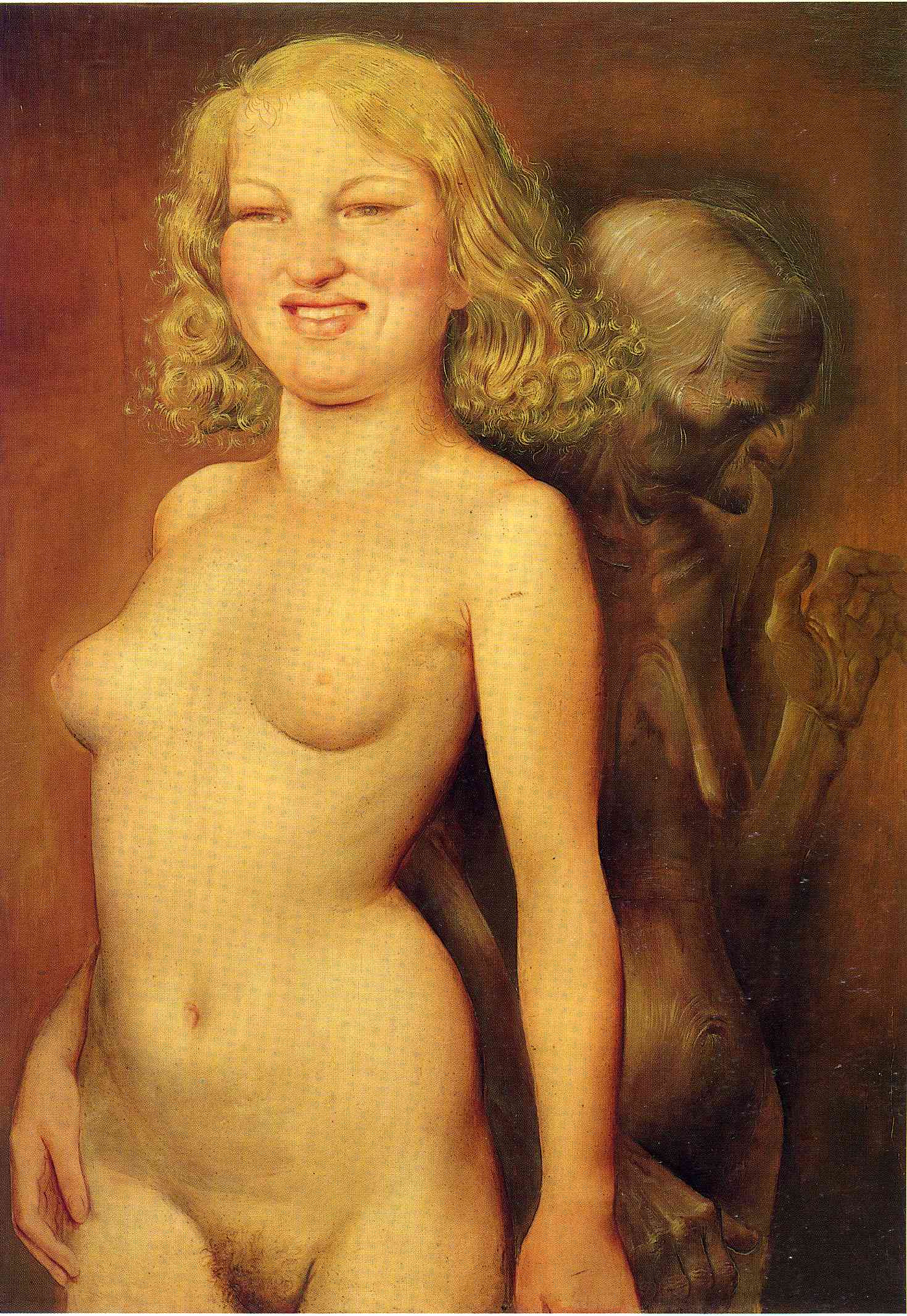This painting features two nude figures prominently displayed against a sepia-toned background that subtly transitions into shadowy obscurity. In the foreground stands a younger woman with golden hair and cherubic features, her bright light and radiant smile strikingly contrasting with the rest of the scene. Her body is fully revealed, and an arm is positioned in front of an older, wearier figure behind her. This older figure, shown in a shadowy, aged state, has a downcast expression and a hand raised, adding an air of solemnity and reflection. Notably, the younger figure's face does not seem to naturally match her body, creating an odd visual flow. The painting lacks any visible autograph, artist signature, or date.